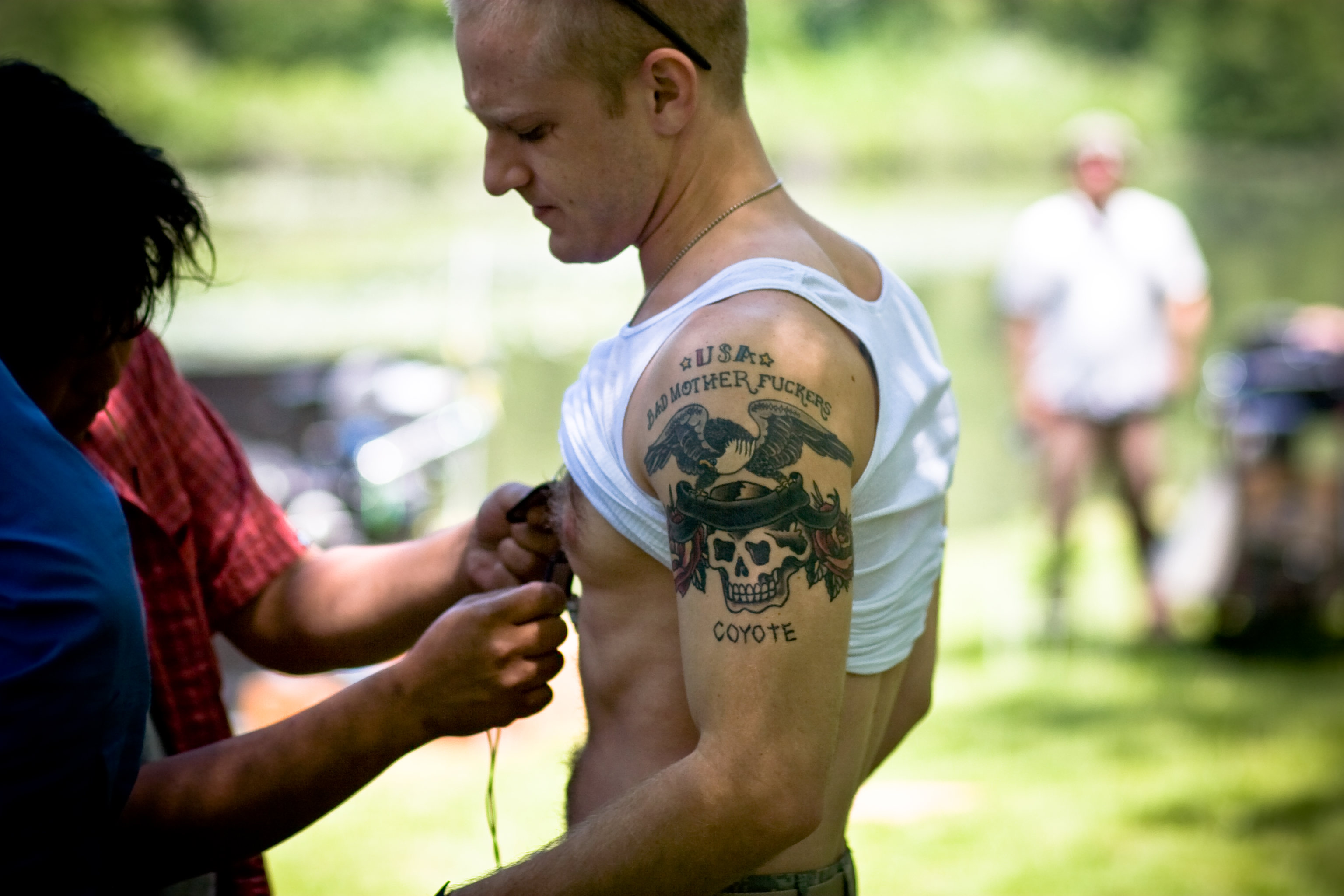The photograph captures an outdoor scene with three individuals. At the center of the image is a man, visible from the waist up, getting wired up for a microphone. The man is wearing a white tank top, pulled up above his chest, revealing a tattoo on his left shoulder that depicts a skull with an eagle perched atop it and the word "Coyote" inscribed below. Additionally, he has "USA" tattooed on his arm. He is seen in a side profile, facing left, with sunglasses on. To the left side, mostly cut off by the edge of the photograph, are two individuals assisting him. The forefront person is dressed in blue, while the rear person is wearing red. The setting appears to be an open field or park with greenery and shrubbery in the background, indicating that it is daytime.